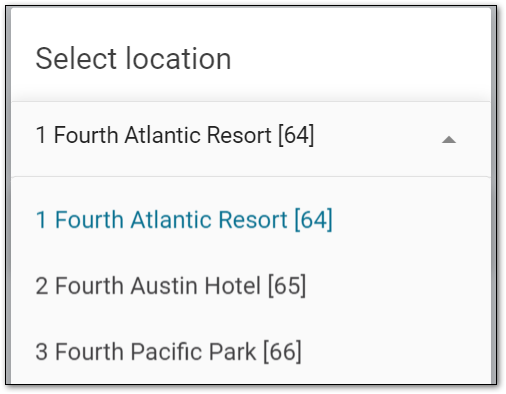A cropped section of a web page showing a small drop-down selection menu titled "Select Location." The menu presents three options: "4th Atlantic Resort," "4th Austin Hotel," and "4th Pacific Park." Each option is notably labeled with the word "4th" spelled out fully as "F-O-U-R-T-H," followed by corresponding unique IDs: "64" for Atlantic Resort, "65" for Austin Hotel, and "66" for Pacific Park. This snippet appears to be part of a hotel booking or selection interface, highlighting different properties under a common brand name, "4th," with locations spread across Atlantic, Austin, and Pacific regions.